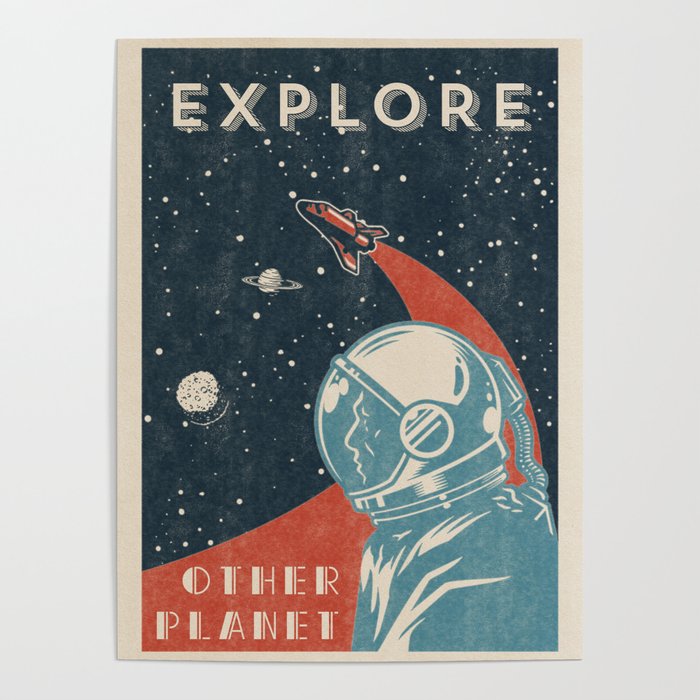The poster features a captivating space-themed design with the word "Explore" prominently displayed at the top and "Other Planet" at the bottom. The background is a deep, star-studded expanse of black space, scattered with numerous white dots representing distant stars. Towards the upper middle section of the poster, a red spaceship is depicted, flying to the left. It leaves a red streak trailing behind it that swoops towards the bottom left corner of the image. To the right of the spaceship, Saturn is easily identifiable with its distinct ring, accompanied by what appears to be a meteor, characterized by a rugged, textured surface. The bottom of the poster showcases the graphic silhouette of an astronaut's profile in either white or light blue, facing left. The entire scene is framed by a clean, white border, all set against a plain white wall background.